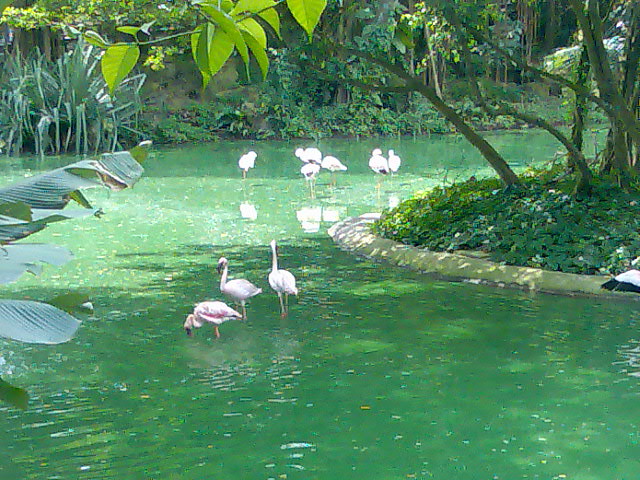The image depicts a serene zoo exhibit featuring a lush, artificial pond filled with murky green water and bordered by dense vegetation. A group of ten flamingos, their pinkish-white plumage reflecting in the water, stands in the pond. Three flamingos are centrally located, bending down towards the water, while six more can be seen farther in the distance, bathing in a patch of sunlight near the pond's curved edge. To the right, a single flamingo is captured mid-motion, its extended wing boasting a striking combination of pink and black feathers. The surrounding oasis is rich with greenery, including dark green banana leaves on the left, palm trees, and a variety of thick, green foliage creating a shaded, tranquil environment. Thin branches and vines stretch upward, adding to the lush atmosphere. The pond curves around a central, overgrown island, which is topped with small trees and multiple shades of green vegetation, including a palm-leaf-like structure extending over the water from the left. The scene is a harmonious blend of wildlife and plant life, evoking a tropical ambiance within the zoo setting.